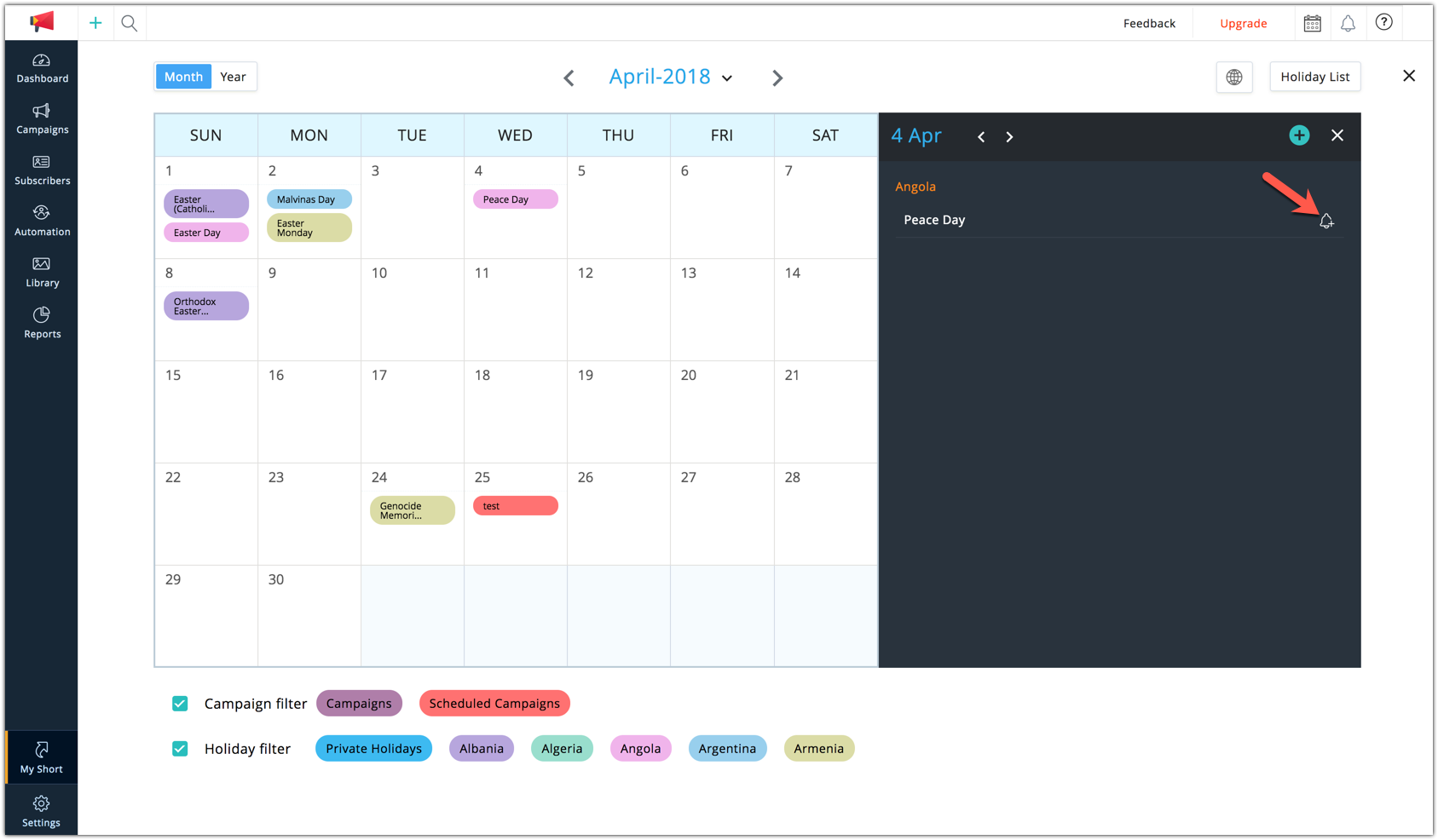The image showcases the face of a digital calendar displaying the month of April 2018. Centrally positioned, the text "April 2018" is written in a light blue font. Flanking the month's title, there are arrows pointing in opposite directions, presumably for navigating between months. The month toggle is marked with a highlighted blue button, while the background of the year toggle is white, appearing unselected or inactive.

On the left-hand corner of the image, there is a vertical sidebar featuring a border filled with various icons and labels. From top to bottom, the sidebar includes icons and text for different sections: "Dashboard" accompanied by an appropriate icon, "Campaigns," "Subscribers," "Automation," "Library," and "Inputs." Towards the bottom of this sidebar, there is a slightly blurred label that appears to read "My Short." Right beneath that is a cog icon followed by the label “Settings.”

The calendar layout itself displays the complete grid for April 2018, featuring the days of the week and individual date squares. Several dates are highlighted with distinct colored ovals; purple and light blue. Notably, there is a light blue oval marking Mother’s Day on Monday, April 2nd.

Along the bottom of the calendar, there are various buttons providing additional functionalities such as "Campaigns,” “Schedule,” "Campaign Button," among others, offering expanded options and information related to the calendar’s primary use.